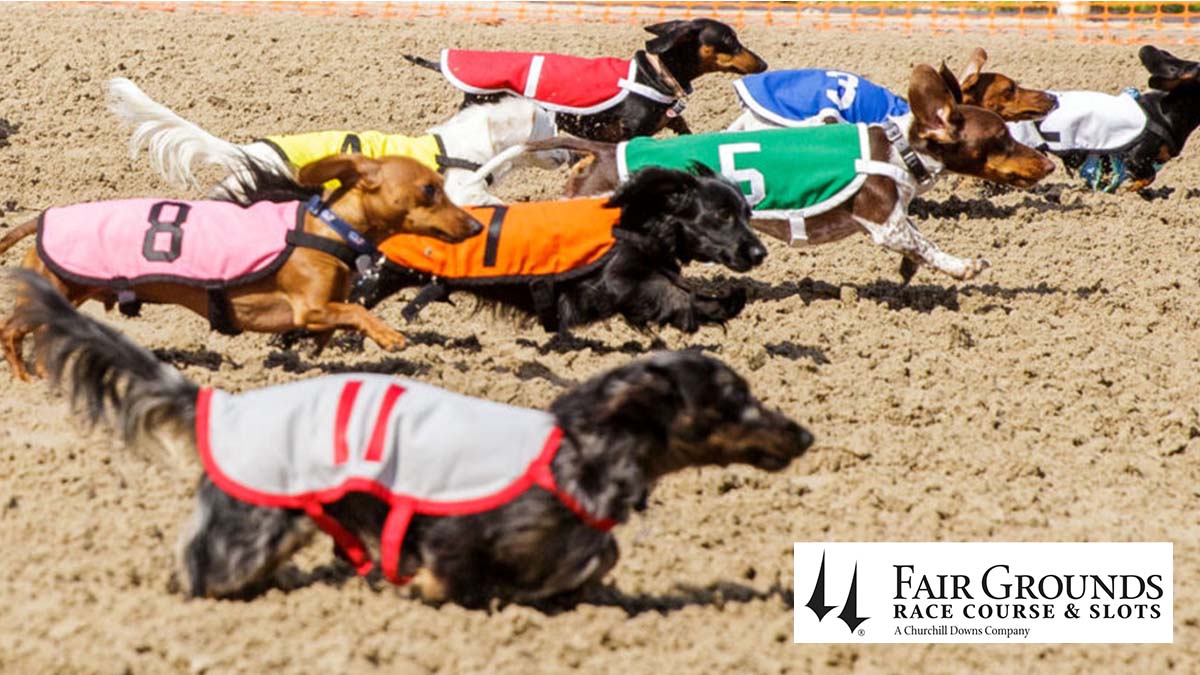The image depicts an exciting dog race held at the Fairgrounds Racecourse and Slots, a Churchill Downs company, prominently displayed in the bottom right corner. The scene captures numerous small dogs, many of which are miniature dachshunds, racing on a sandy dirt track reminiscent of a horse racing track. Each dog is adorned with a colored strap featuring a unique number, much like jockey silks, with the number 11 dog in a red strap taking the lead. Behind it, other dogs sporting numbers 8 to 1 in various colors, such as pink, orange, green, yellow, blue, and white, gallop along the tilled soil. Notably, one dog has short brown hair, another has longer black hair, and a distinctive one has a white-spotted leg, adding to the vibrant diversity of the participants.